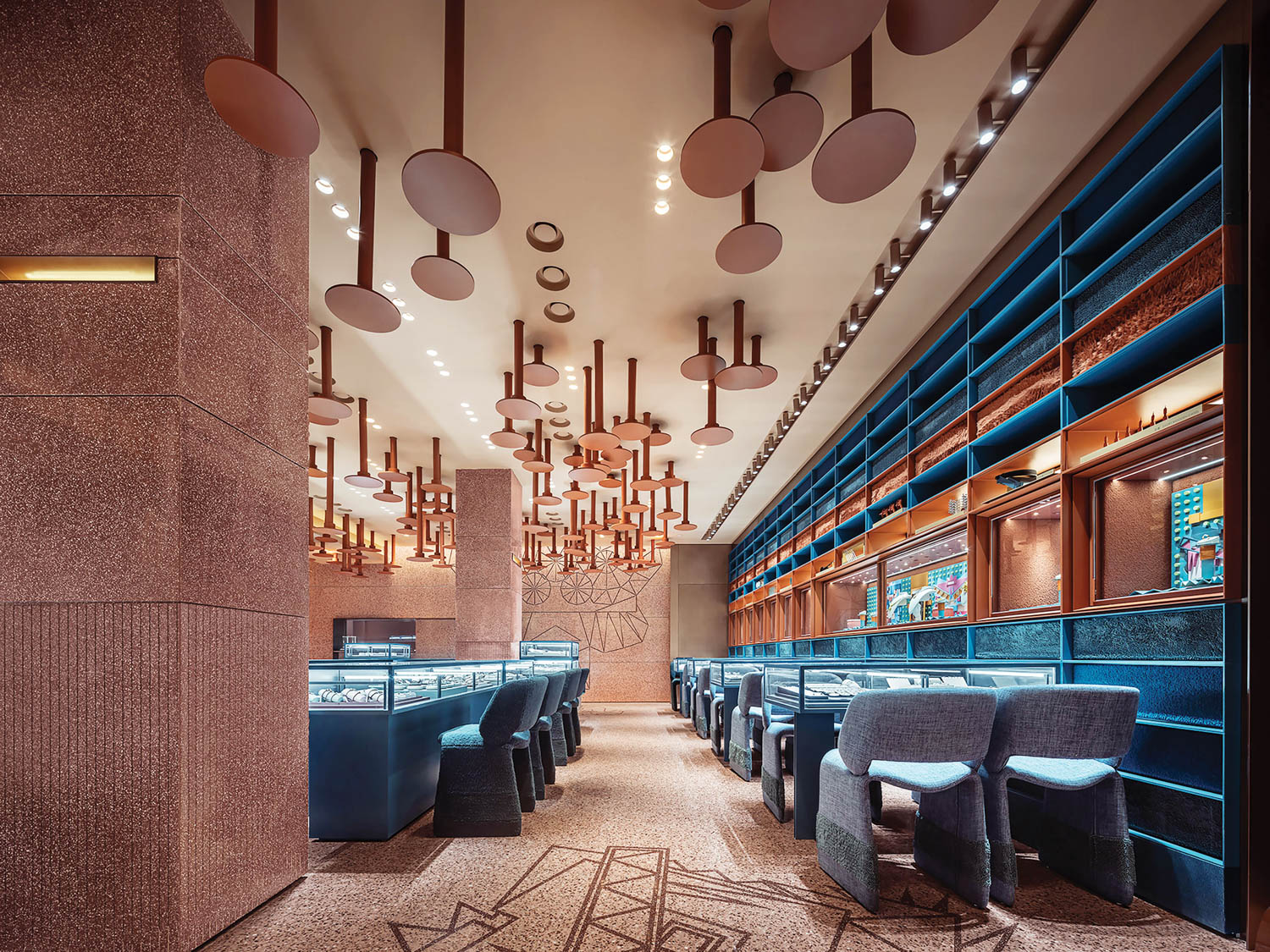This image appears to be an AI-generated depiction of a high-end, eclectic jewelry store. The store features a modern and artistic design with gray carpeting adorned with intricate patterns which extend onto the walls. Display cases filled with jewelry are strategically placed on both the left and right sides of the room, each flanked by gray, cushioned slide-out chairs. 

The ceiling is a notable highlight, showcasing an array of artistic fixtures resembling mushrooms with flat, circular tops suspended on metal rods at varying heights. These fixtures are complemented by recessed lighting, contributing to a futuristic ambiance. 

Against the right wall, there is a sequence of glass cases showcasing additional jewelry items, providing a sleek and functional display setup. Above these cases are blue and brown drawers, possibly used for storage or as a design element. The same pattern from the carpet is also present on the back wall, providing a cohesive aesthetic. Gray columns are dispersed throughout the space, serving as structural supports and adding to the overall sophisticated feel of the store.